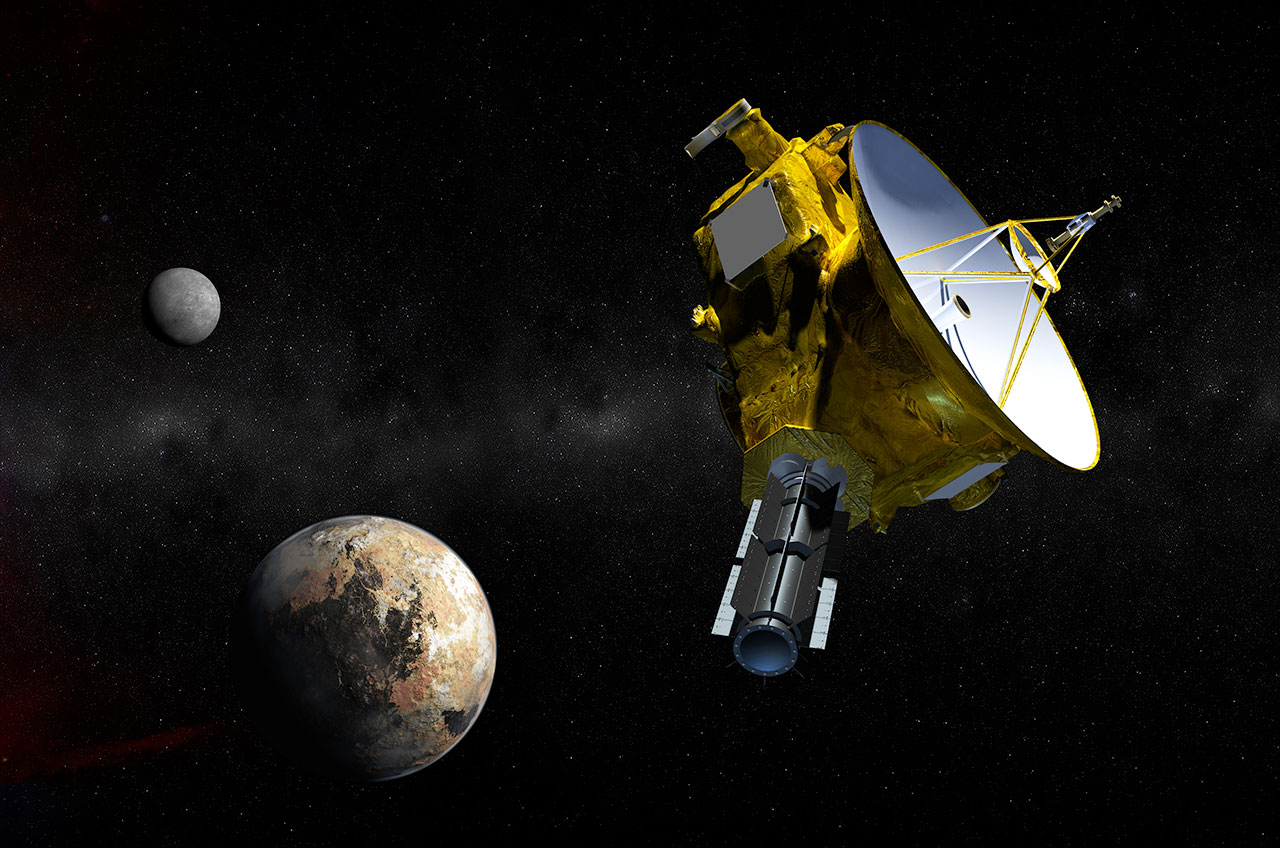In this detailed 3D-rendered image of outer space, a scene unfolds featuring a large, predominantly gold-colored satellite with a white dish at its center, precariously covered in green gook. The satellite's intricate structure includes wires and a frame that connect to a smaller, signal-transmitting unit positioned on top. A conspicuous black cannon protrudes from its edge. The cosmic backdrop reveals a tapestry of stars scattered across the black canvas, with a partially illuminated gray moon on the left. Below it, a planet resembling Earth is depicted, albeit in an unnatural palette of brown and white hues, diverging from its usual blue and green. In the distant background, another planet can be discerned, completing the celestial vista.